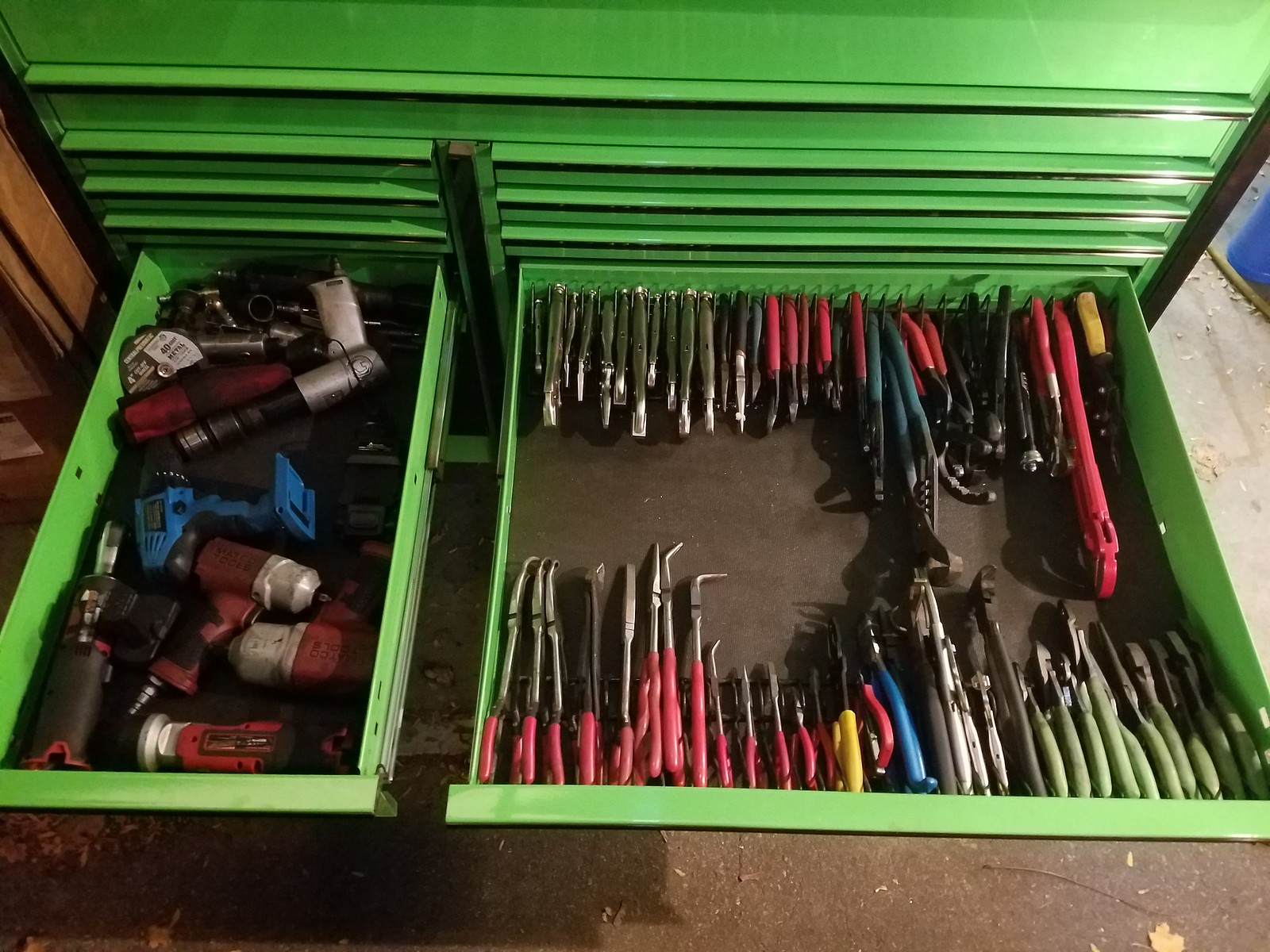This image captures a well-organized green metallic tool cabinet, likely situated in a tool shop or garage with a concrete floor. The cabinet, which appears to be quite tall—nearly six feet—is equipped with numerous thin, rectangular drawers, of which two are extended. Each drawer features a black strip. The bottom drawer of the unit, divided into a wide right section and a narrower left section, showcases an array of neatly arranged tools. On the right, the larger compartment contains various wrenches and drills orderly positioned, some facing downwards. The tools exhibit a color-coded scheme with red-handled tools at the bottom, green-handled ones to their left, and drills towards the top. The left section houses more compact tools and different types of augers, efficiently utilizing the space by placing tools against the walls, leaving the center clear. The photo, taken from an elevated angle, provides a comprehensive view of the meticulous arrangement, highlighting the functional and organized nature of the tool cabinet.